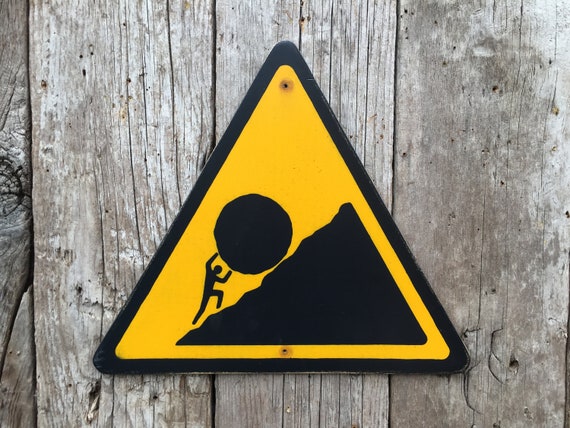The image depicts a triangular metal warning sign with a black border and a bright yellow interior. Inside the triangle, in stark black, is a silhouette of a stick figure man pushing a large boulder uphill on a slope, evoking the myth of Sisyphus. The man appears to be in the motion of pushing the boulder with one knee up. This sign is affixed to a backdrop of weathered wooden planks, which exhibit a mix of colors including desaturated dark brown, lighter brown, and white. The wood appears aged and distressed, suggesting the location could be an outdoor area such as a balcony, shed wall, or fence.